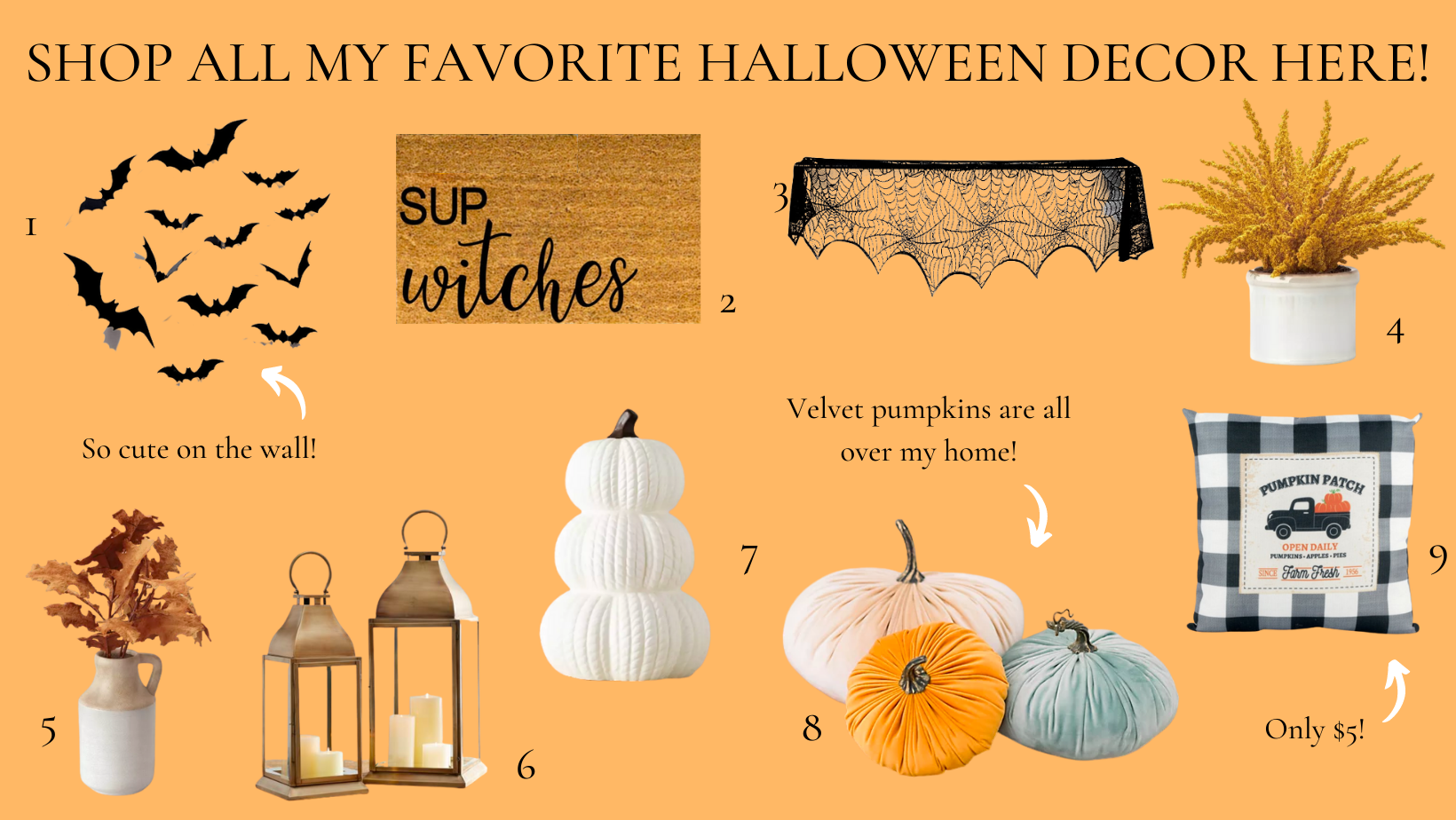**Detailed Description: Festive Halloween Decor Advertisement**

The advertisement features a bold, plain orange background that unmistakably sets the tone for the Halloween season. The header reads, in striking black text, "Shop all my favorite Halloween decor here."

Highlighted within the advertisement are nine distinct Halloween decor items:

1. **Bat Wall Stickers**: Located on the left side of the image, these bat-shaped stickers are described as "so cute on the wall." They come in a pack of approximately ten and are perfect for adding a spooky touch to any room.

2. **'Sup' Doormat**: To the right of the bat wall stickers is a simple yet inviting brown doormat that says "sup," a casual short form of "what's up." It offers a laid-back greeting for any front door.

3. **Spider Web Curtain**: Below the doormat, a black curtain adorned with intricate spider web designs adds a subtle yet eerie ambiance to any window or doorway.

4. **Autumn Plant Holder**: This plant holder, with a plant resembling wheat, sits next to the spider web curtain. Its autumnal theme brings a touch of fall indoors.

5. **Autumn Leaf Pitcher**: Positioned on the next row, this white pitcher is artistically filled with vibrant orange and brown autumn leaves, perfect for a seasonal centerpiece.

6. **Glass Lanterns**: Beside the pitcher, a set of glass lanterns with light brown tops frame plain white candles, casting a warm, inviting glow.

7. **Pumpkin Snowman**: A whimsical decoration featuring three white pumpkins stacked on top of each other, similar to a snowman, adds a playful touch to your decor.

8. **Velvet Pumpkin Pillows**: These pumpkin-shaped and colored pillows, described as "velvet pumpkins," are cozy additions to your living space. An arrow points to them with the text "velvet pumpkins are all over my home."

9. **'Pumpkin Patch' Pillow**: A square black and white plaid pillow with an illustration of a vintage truck carrying pumpkins, labeled "pumpkin patch." Below the truck reads "only five dollars." This pillow also has an arrow directing attention to it.

Each item is meticulously showcased, inviting viewers to explore and select their favorite pieces to bring the Halloween spirit into their homes.